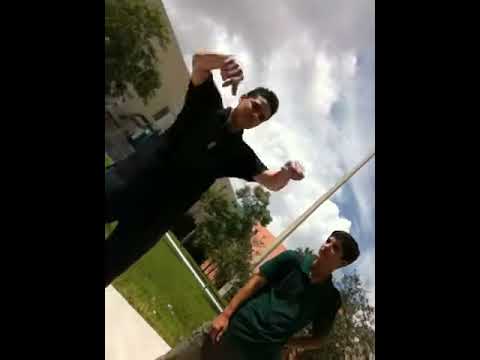The photograph captures two young teenagers, one wearing a green polo shirt and pants, the other dressed in a black shirt and pants, in a slightly askewed or tilted angle shot, lending a Dutch angle effect. The teenager in the green shirt, who appears to be either white or Hispanic with dark hair, is intently looking at his friend on his right. His friend, a black or brown-skinned teenager with black hair, is animatedly holding his hands up as if mimicking the act of revving a motorcycle. They are standing on a well-manicured concrete walkway within a park or school area. The background reveals an expanse of green grass, large buildings, and a tall pole that may be a flagpole or streetlight stretching into the sky. The day appears overcast yet sunny, with clouds visible against the blue sky. The photograph is grainy and somewhat blurry, suggesting it was taken with an older camera, and features black bands on both sides, indicating it might have been taken in portrait mode on a cell phone.